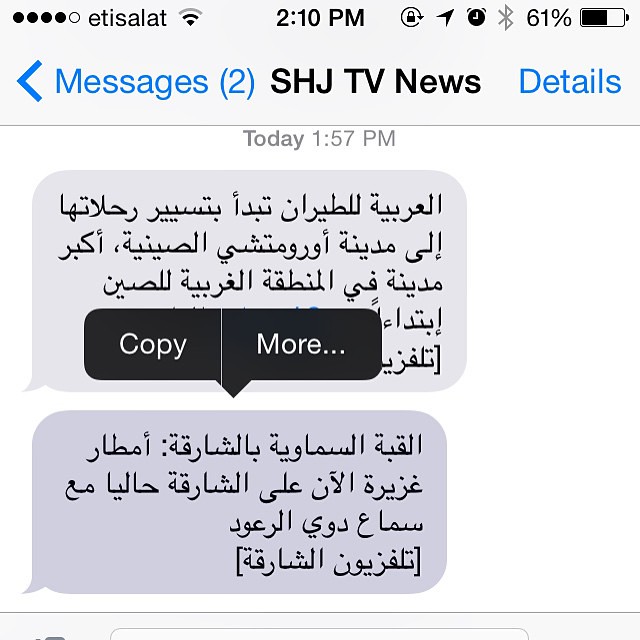This screenshot captures a chat in a messaging app on a mobile phone, indicating the phone's current status and app details. At the top of the image, the notification bar displays an array of symbols including Wi-Fi, time (2:10 PM), a lock, Bluetooth, and a battery level at 61%. Below, the app bar presents options labeled "Messages (2)," "SHJ TV News," and "Details." The main content features two text bubbles that appear to be in Urdu, timestamped 1:57 PM with an annotation "Today." The background of the text messages is light grey, while the general background is white. A "Copy" and "More" option is visible next to the text bubbles, suggesting ongoing interaction with the message, possibly for translation or other purposes. The name "Etis Alat" is also noted at the top, likely referring to the service provider or network.